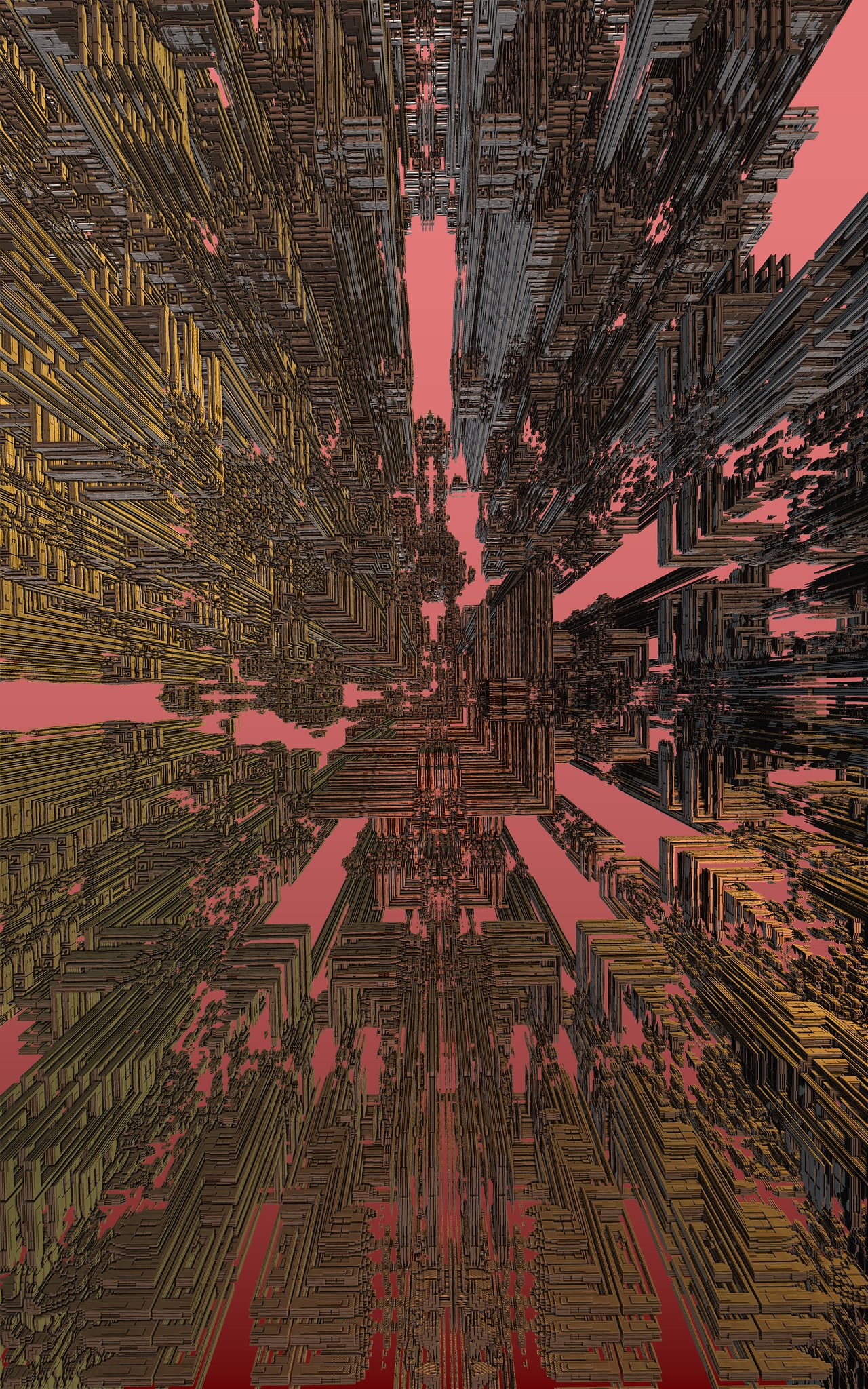The image appears to be a piece of modern or computer-generated artwork, presenting an intricate and abstract scene. The background transitions from light pink at the top to dark red at the bottom, creating a gradient that resembles a salmon hue. This vibrant backdrop is partially obscured by a complex web of brown geometric lines, evoking the impression of numerous pipes or tunnels. These lines give the illusion of depth, as if one is peering into an elaborate underground network or between towering skyscrapers that stretch into the distance. The top corners of the image showcase lighter shades, transitioning to darker tones towards the center and bottom, where the salmon background becomes more visible. The overall effect is one of dynamic movement, as though the viewer is being pulled through the scene at high speed.